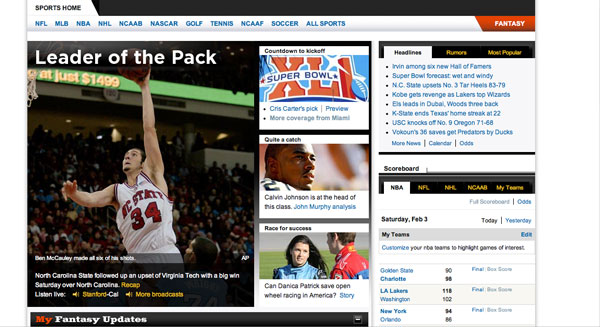In the image, the webpage prominently features a main section dedicated to various sports categories, listed at the top as NFL, MLB, NBA, NHL, NCAAB, NASCAR, golf, tennis, NCAAF, soccer, and a catch-all category labeled "all sports." On the left side of the main content area, an action shot captures an NC State player, wearing jersey number 34, leaping upward, either to catch the ball or block it. This intense moment is highlighted as "Leader of the Pack." On the right side of this main section, columns filled with articles and information about other sports are displayed. The background of the main image reveals a packed stadium with fans filling the seats, adding to the electrifying atmosphere. Adjacent to the main picture, a block marked "XL1" indicates content related to the Super Bowl. While much of the print in this section is too small to decipher, it appears to include team stats positioned at the bottom right corner.